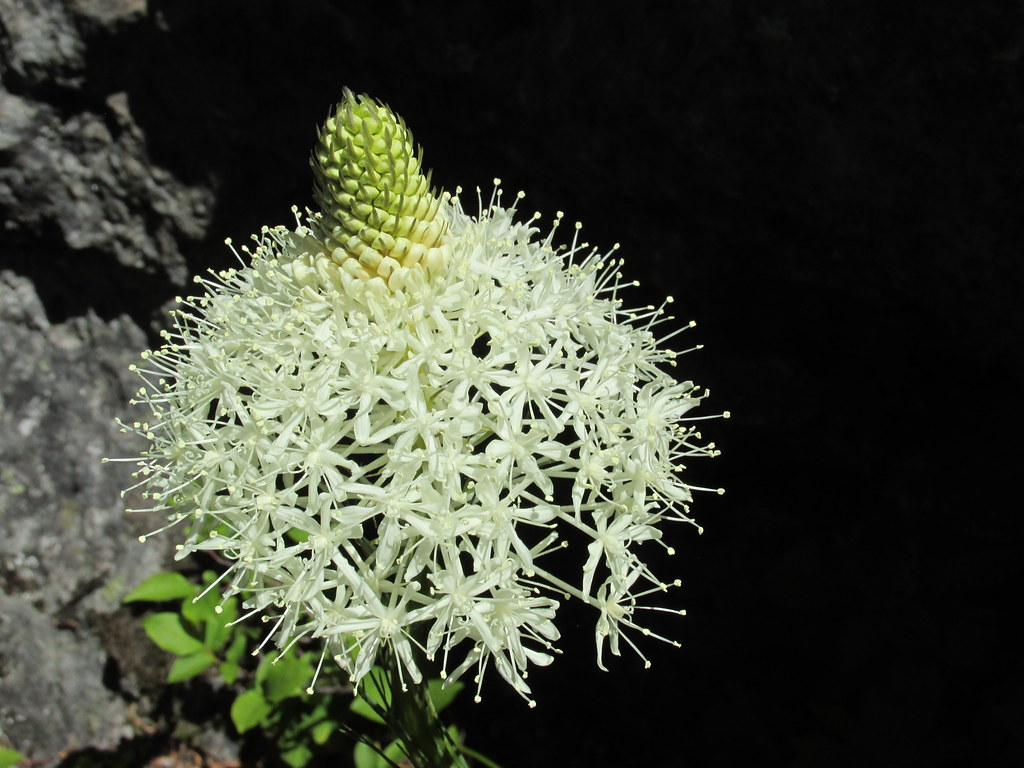This image is a detailed close-up photograph of a flowering plant against a dark, blurry background. The centerpiece is a striking cluster of small, star-shaped flowers with a unique bowl-shaped arrangement. Each individual flower in the cluster has five to six creamy white petals that radiate from a bright yellow center, resembling spokes. Tiny, slender filaments emerge from the petals, further accentuating the star-like appearance. At the heart of the cluster is a notable cob-like protrusion that transitions from green to white. Surrounding this central feature, some green, waxy leaves and possibly blurred gray rocks are faintly visible in the periphery, adding a touch of natural context to the pristine floral display. The overall composition and the black background emphasize the intricate details of the flowering plant, making it stand out beautifully.